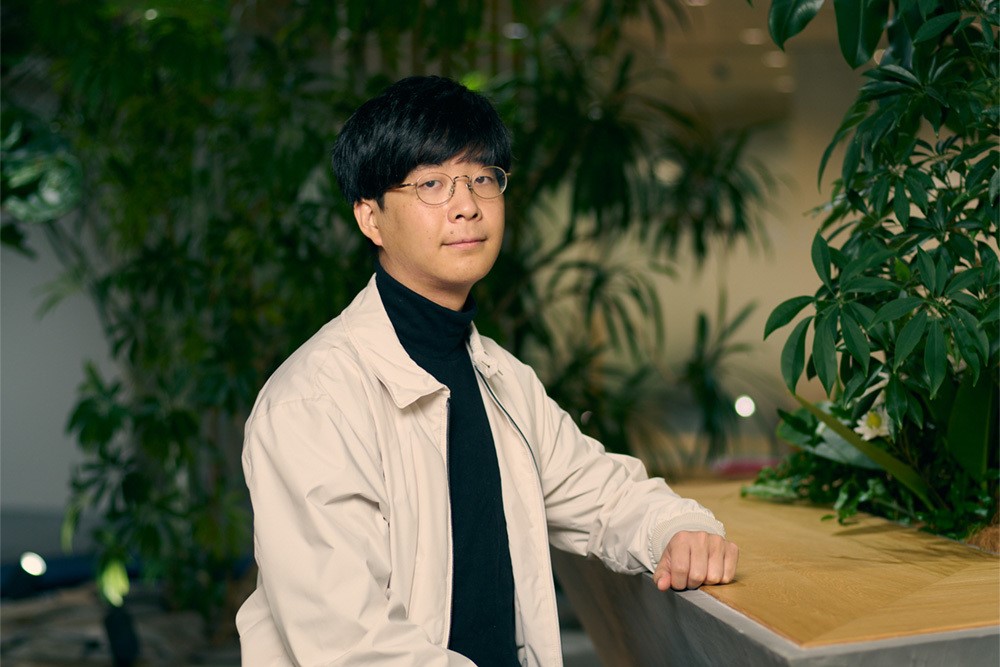This is a detailed landscape-mode, photorealistic portrait of an Asian man, shot from about the waist up. He is wearing round glasses and sporting a bowl cut reminiscent of the 60s. His attire includes a black turtleneck, covered by a light cream or beige-colored jacket. The man's expression is neutral as he gazes directly at the camera. His left arm rests on a wooden countertop with gray sides, while a lush, leafy plant is prominently positioned to his right. The out-of-focus background features more green plants and blurred lights, enhancing the natural and serene atmosphere of the scene.